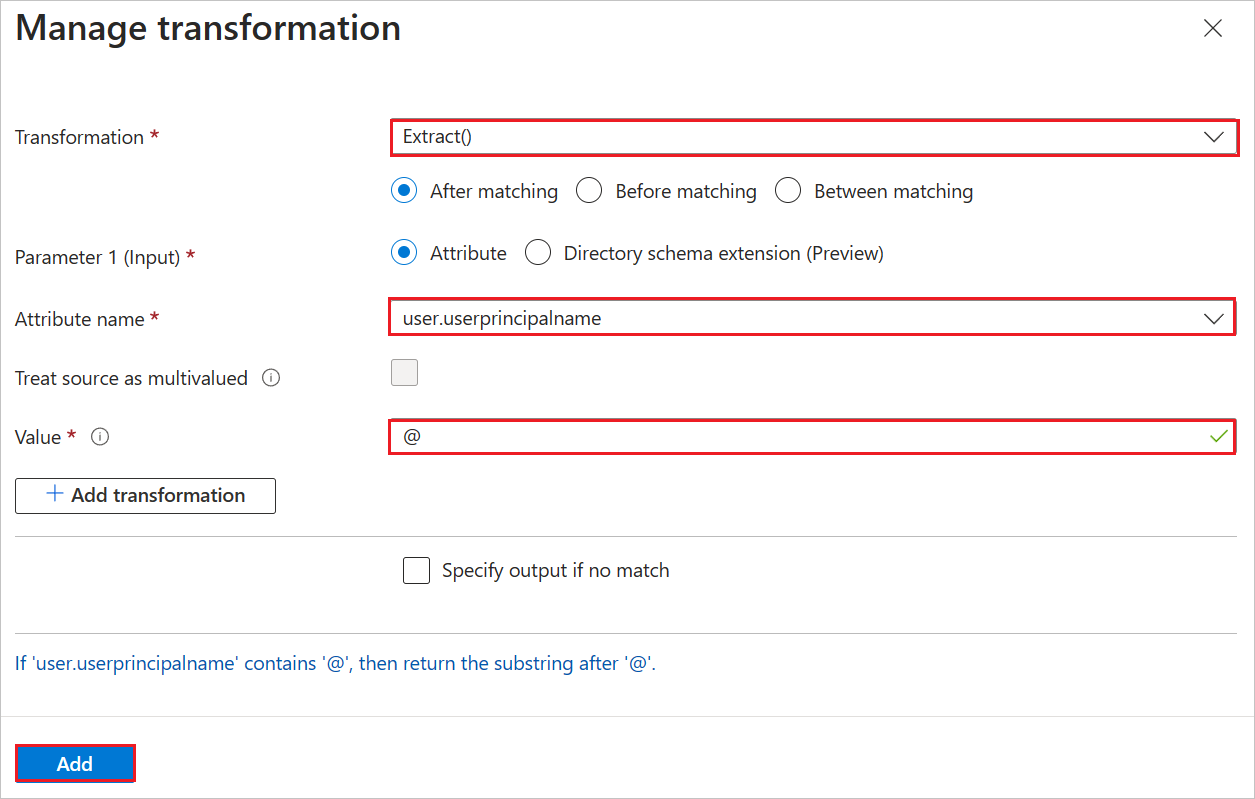The image displays a user interface for managing transformations, with detailed options and selections. Here's an organized and descriptive caption:

---

The interface, titled "Manage Transformation," is visible at the top left corner. Beneath the title, there is a heading labeled "Transformation," marked with a red star icon. Under this, a red box with black text reads "Extract," accompanied by a down arrow icon.

Below the "Extract" option are four radio buttons for sequence settings: "After Matching," "Before Matching," "Between Matching," and one more. The "After Matching" option is selected.

Moving further down, there is a parameter labeled "Parameter 1 (Input)," indicated by a red star icon, with two sub-options: "Attribute" and "Directory Schema Extension (Preview)." The "Attribute" option is chosen.

Next, the interface displays the field "Attribute Name," marked by a red star icon. A red box contains the text "user.userPrincipalName."

Further down, the interface mentions "Tree Source as Multivalued," with an informational "i" icon in a gray circle. This option includes a checkbox that is not checked.

Below this, there is a field labeled "Value," with a red star icon and another informational "i" icon. Inside a red box, the text "@ domain.com" is displayed, and a green check mark appears on the far right of the box.

Under these settings, there are buttons for "Add Transformation" and another one labeled "Add Transformation" again, each enclosed in a gray-bordered box. A horizontal gray line spans from left to right between these buttons.

Additionally, there is an unchecked checkbox labeled "Specify Output if No Match," followed by another horizontal gray line.

Towards the bottom of the interface, a blue text reads, "If user.userPrincipalName contains '@' then return the substring after '@'." This statement is framed within a red-bordered blue box, which includes an "Add" button in white text, completing the detailed transformation options interface.